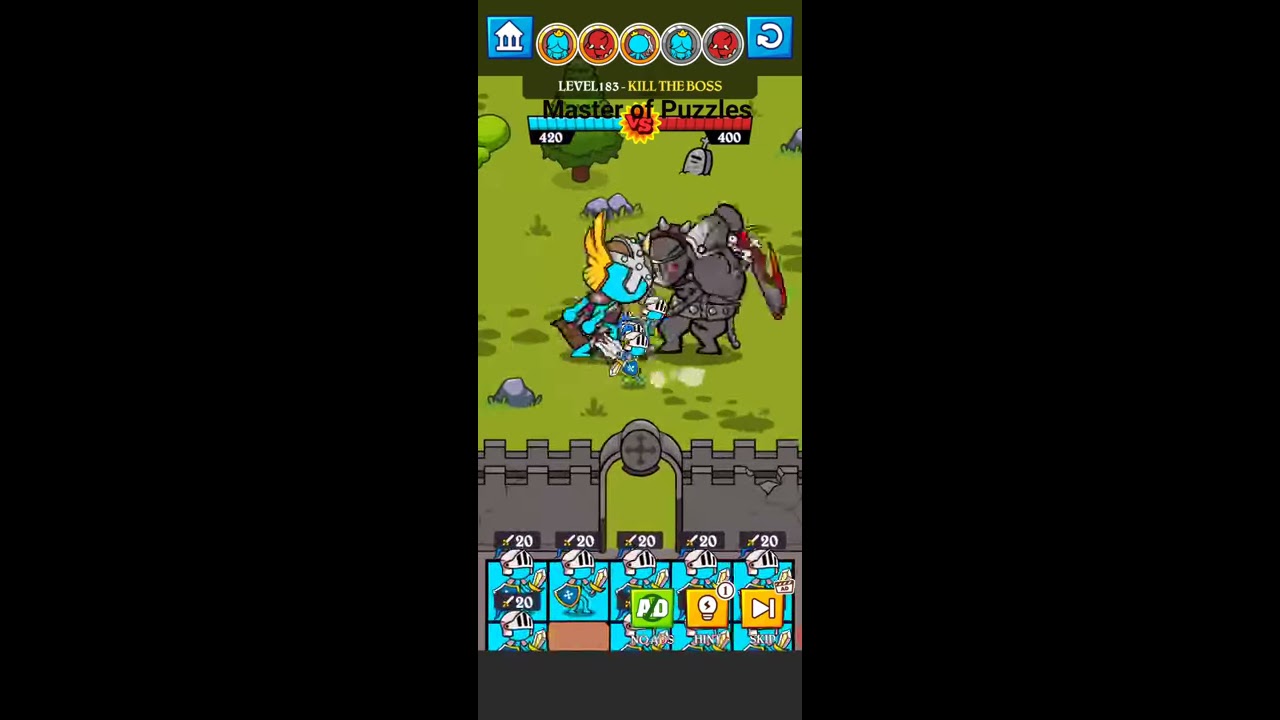This is a detailed screenshot of a phone app video game featuring a battle scene. The central visual shows two armored characters, one in blue with silver and brown helmet adorned with gold wings, and the other in gray with red accents, engaged in combat on a ground covered with lush green grass and scattered stones. They are positioned in front of a dark gray castle wall with an opening. Surrounding the combat scene is a natural setting, complete with a green tree.

At the top of the game screen, a horizontal bar displays various game interface elements. On the left, there is a home button icon, while on the right, there is a reverse icon. In the middle, five character icons are arranged in a row, with text beneath them reading "Level 183 - Kill the Boss" and "Master of Puzzles." Below the main battle scene, the health meters for each character are visible, with the blue character's health at 420 and the red character's health at 400.

Additional game control icons are seen at the bottom of the screen, likely used to manage the characters in combat. The entire game interface is contained within a central rectangular frame against a black background, resembling the screen of a smartphone. The vibrant colors and detailed setting create an immersive and engaging game experience.